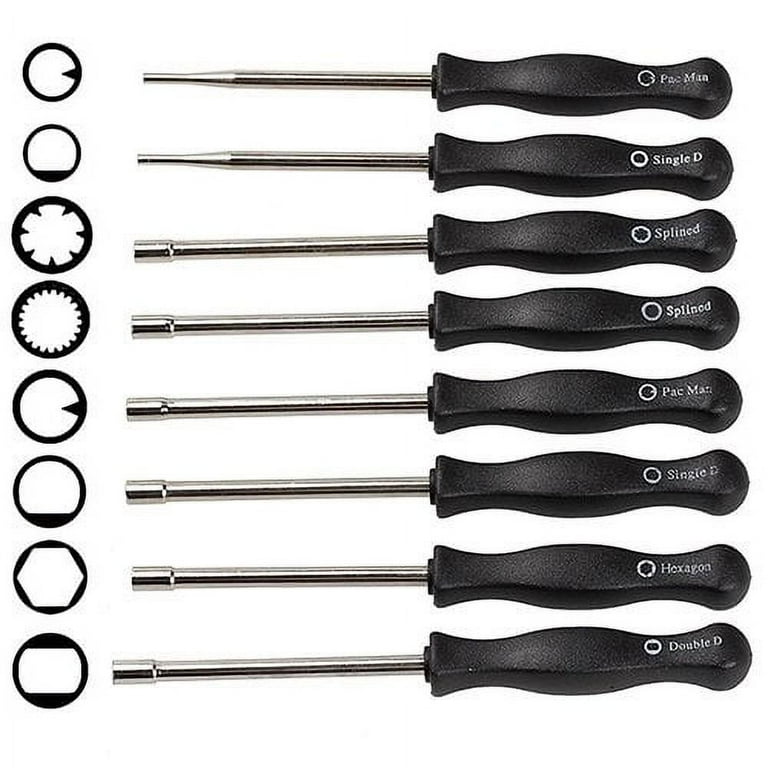The image features a set of seven nut driver tools aligned vertically, each with a black plastic handle and a metal shaft resembling a screwdriver but with unique driver shapes. Each tool is labeled from top to bottom as Pac-Man, Single-D, Splinod, Hotsport, and Double-D. They are stacked horizontally with the handles on the right. On the left, detailed illustrations depict the distinctive shapes of the corresponding driver sockets, including configurations such as a circle with a triangular point, a circle with a solid black base, and a circle with jagged teeth in the center.